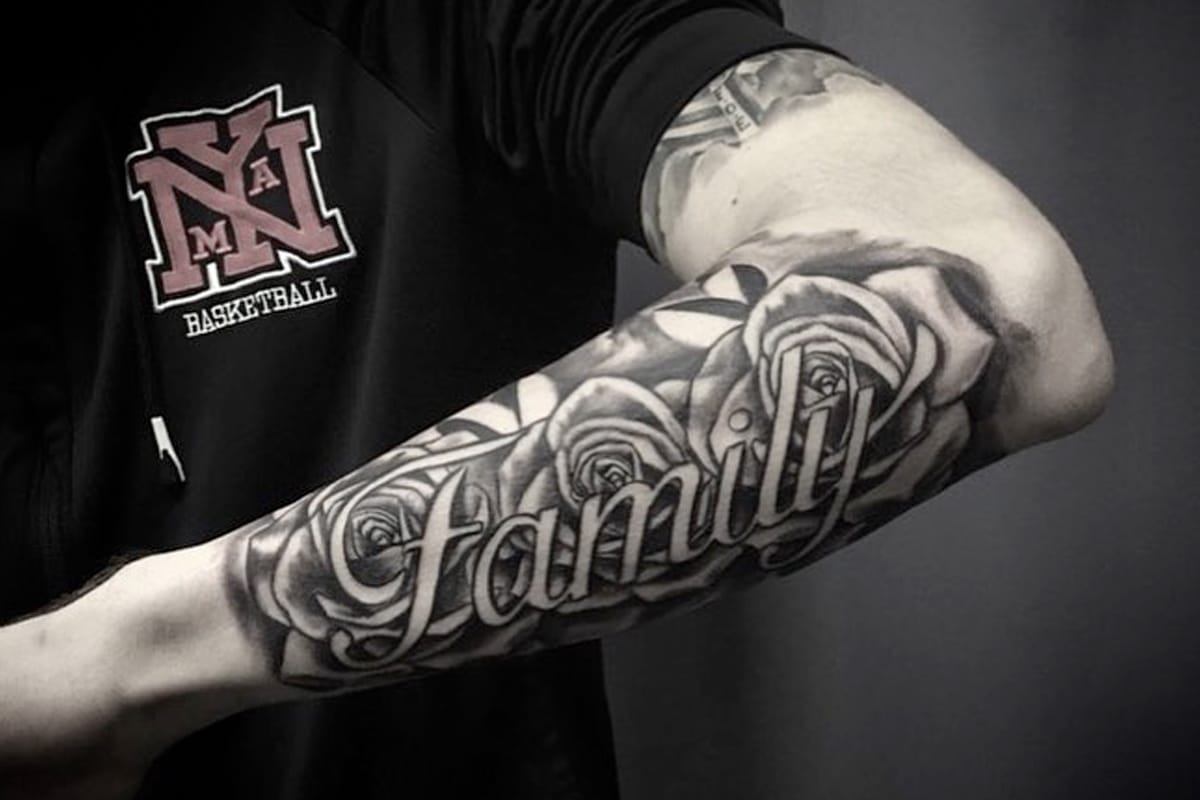In the photograph, a close-up of a man’s bent left arm is shown against a dark background. The man’s forearm is prominently featured, adorned with an intricate black-and-white tattoo of three roses and the word "family" elegantly scripted in a fancy white cursive font. Just visible beneath the rolled-up sleeve of his black athletic top is the beginning of another tattoo on his upper arm, mostly obscured by the fabric. The distinctive athletic shirt bears a pink logo on the chest consisting of the letters "N" and "Y" with smaller "M" and "A" inside, followed by the word "basketball" in white letters. The partial view of his hand is directed towards the lower left corner of the image, while the overall scene is set against a subdued, almost monochromatic background perhaps highlighting the subtle red in the logo.